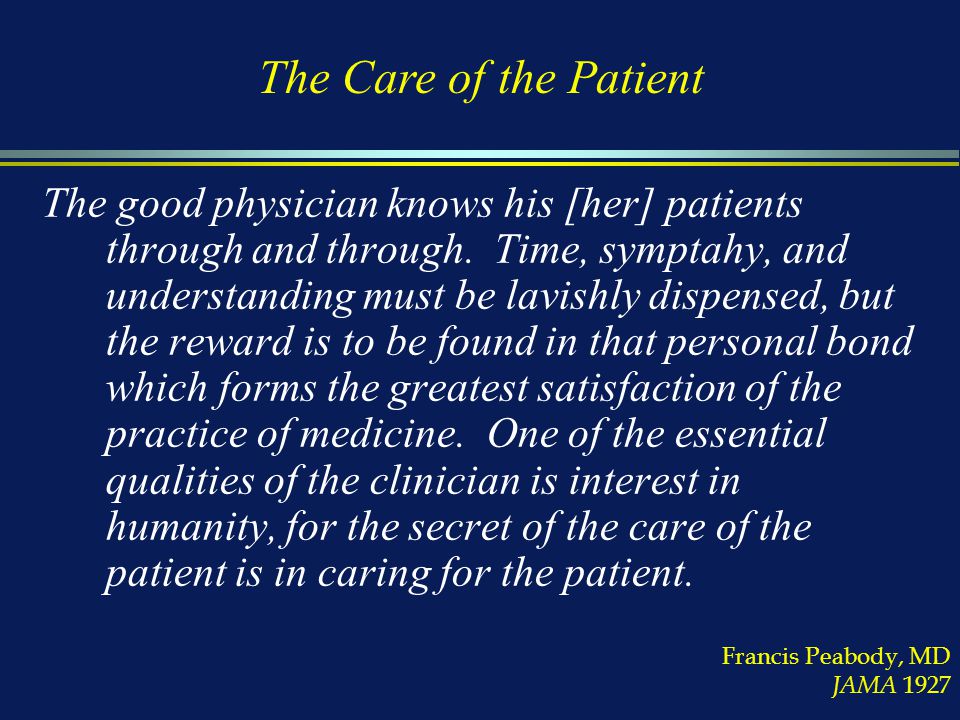The image is a digital slide with a navy blue background, featuring the title "The Care of the Patient" in yellow text at the top. Beneath the title, there are two thin, horizontal lines—one white and one yellow. The rest of the text is in white and contains a quote by Francis Peabody, M.D. from JAMA, 1927. The quote reads: "The good physician knows his or her patients through and through. Time, sympathy, and understanding must be lavishly dispensed, but the reward is to be found in that personal bond, which forms the greatest satisfaction of the practice of medicine. One of the essential qualities of the clinician is interest in humanity, for the secret of the care of the patient is in caring for the patient." In the lower right-hand corner, his name and the publication details are repeated: "Francis Peabody, M.D., JAMA, 1927".